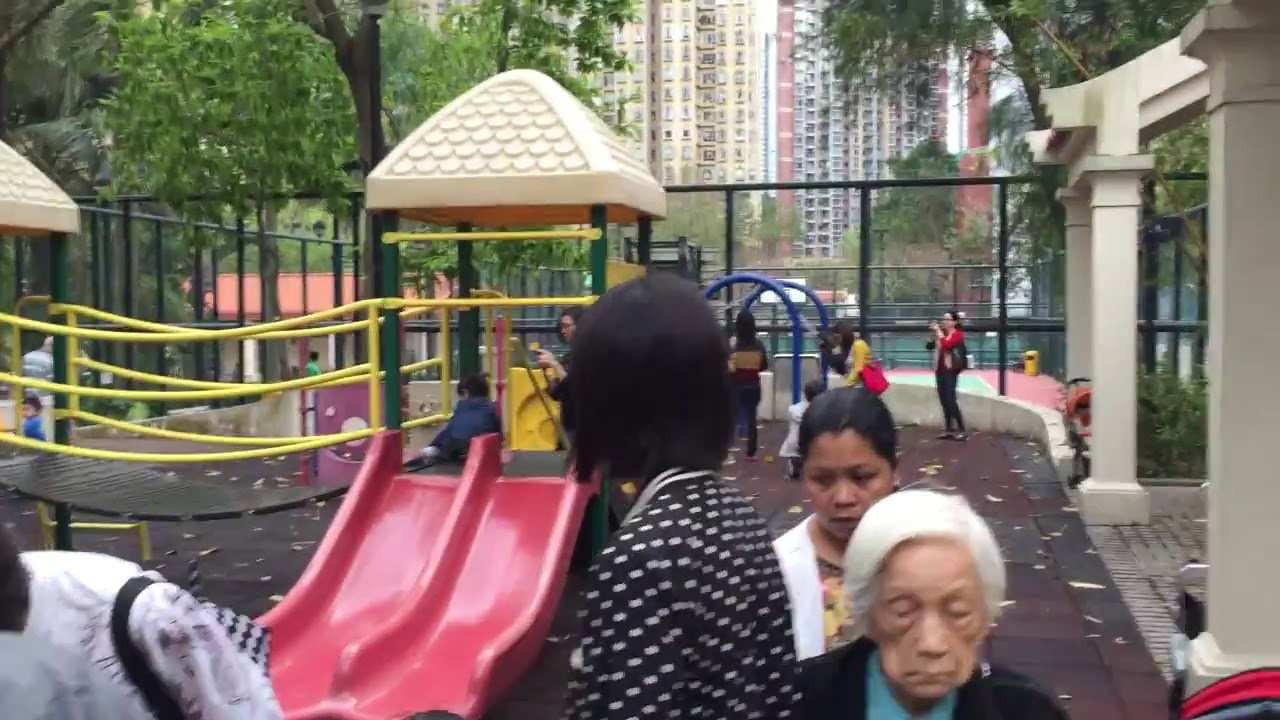The image depicts a rainy day at a city playground, characterized by wet red brick ground. The playground, surrounded by a likely chain-link fence, features vibrant play structures, including a double red slide, a plastic slide for young children, a wooden-slatted crossing bridge, and various climbing fixtures. Beyond the playground, there is a body of water, possibly a canal, and residential high-rises, trees, and other structures.

In the foreground, several Asian women of varying ages are visible. One notably elderly woman, likely in her 80s, with short white hair and wrinkled skin, wears a black cardigan over a blue dress. Near her, a middle-aged woman with dark brown skin and dark brown hair, dressed in a white dress, stands alongside another woman with short black hair in a black polka-dotted dress, who has her face turned away.

In the playground, children play under the watchful eyes of adults. A woman wearing a white dress with a purse slung across her shoulder is bending near the slide. Another woman in a red top and black pants, with a black bag on her shoulder, is seen, as well as a lady in a yellow dress with a red bag and long hair. In the background, more women, likely mothers, are engaged with their children on the play structures, with some standing on the bridge and near the monkey bars. The overall atmosphere is vibrant yet serene, despite the rain.